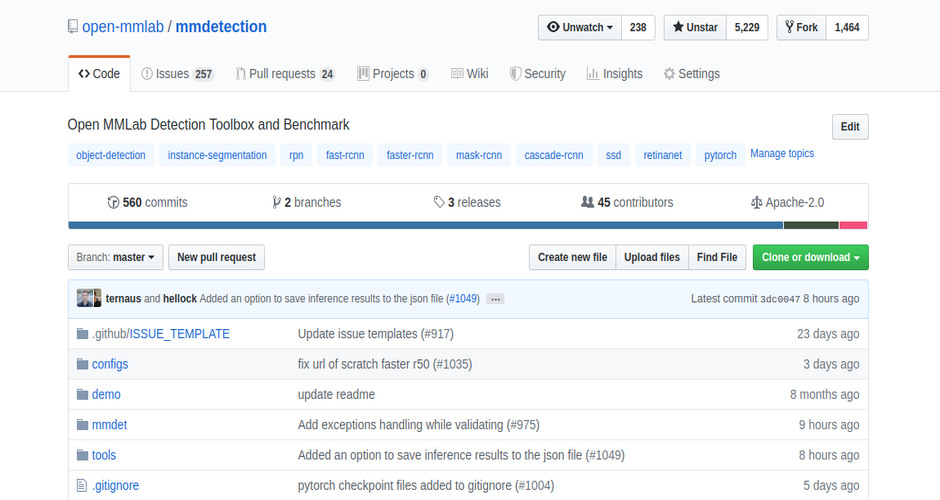This image is a detailed screenshot of the "open-mmlab/mmdetection" repository on GitHub. The repository’s name "open-mmlab/mmdetection" is prominently displayed in the top-left corner. In the top-right corner, the user interface options include "Unwatch" with a dropdown menu, "238," "Unstar" with "5229," and "Fork" with "1464."

At the top of the page, a navigation bar lists several categories: "Code," "Issues," "Pull requests," "Projects," "Wiki," "Security," "Insights," and "Settings." The "Code" tab is currently selected. Beneath this navigation bar, the repository description reads "Open MMLab Detection Toolbox and Benchmark," followed by a series of hyperlinks for different functionalities and modules. These hyperlinks, listed from left to right, include: "Object Detection," "Instance Segmentation," "RPN," "Fast R-CNN," "Faster R-CNN," "Cascade R-CNN," "SSD," "RetinaNet," and "PyTorch," with an "Edit" button directly above that section.

Further down, the repository stats are displayed, indicating "560 comments," "2 branches," "3 releases," "45 contributors," and the license type "Apache 2.0." Below these statistics, a dropdown menu offers options such as "Pull requests," "Create new file," "Upload files," "Find files," and "Clone or download."

Finally, the main content of the page features a list of various files and templates, each clickable, allowing users to navigate through the repository contents.